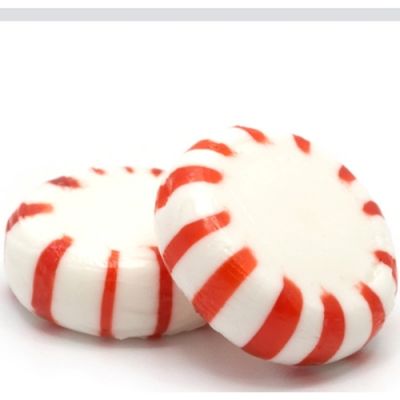This image presents a close-up of two traditional peppermint candies, often recognized as peppermint pinwheels, against a stark white backdrop. Both mints are glossy white with evenly spaced red stripes circling their edges. The peppermint on the left lies flat, viewed from the top left angle, offering a clear perspective of both its top and side. The peppermint on the right overlaps approximately 40% of the mint on the left's right side, leaning at an angle reminiscent of the 4:30 or 5 o'clock position. This composition creates a shadow on the plain white surface, hinting that the light source is positioned from the top right. The image is likely intended for product display, with a very thin gray bar along the top which might serve as a framing element. The peppermints appear glossy, with light reflections enhancing their three-dimensional appeal.